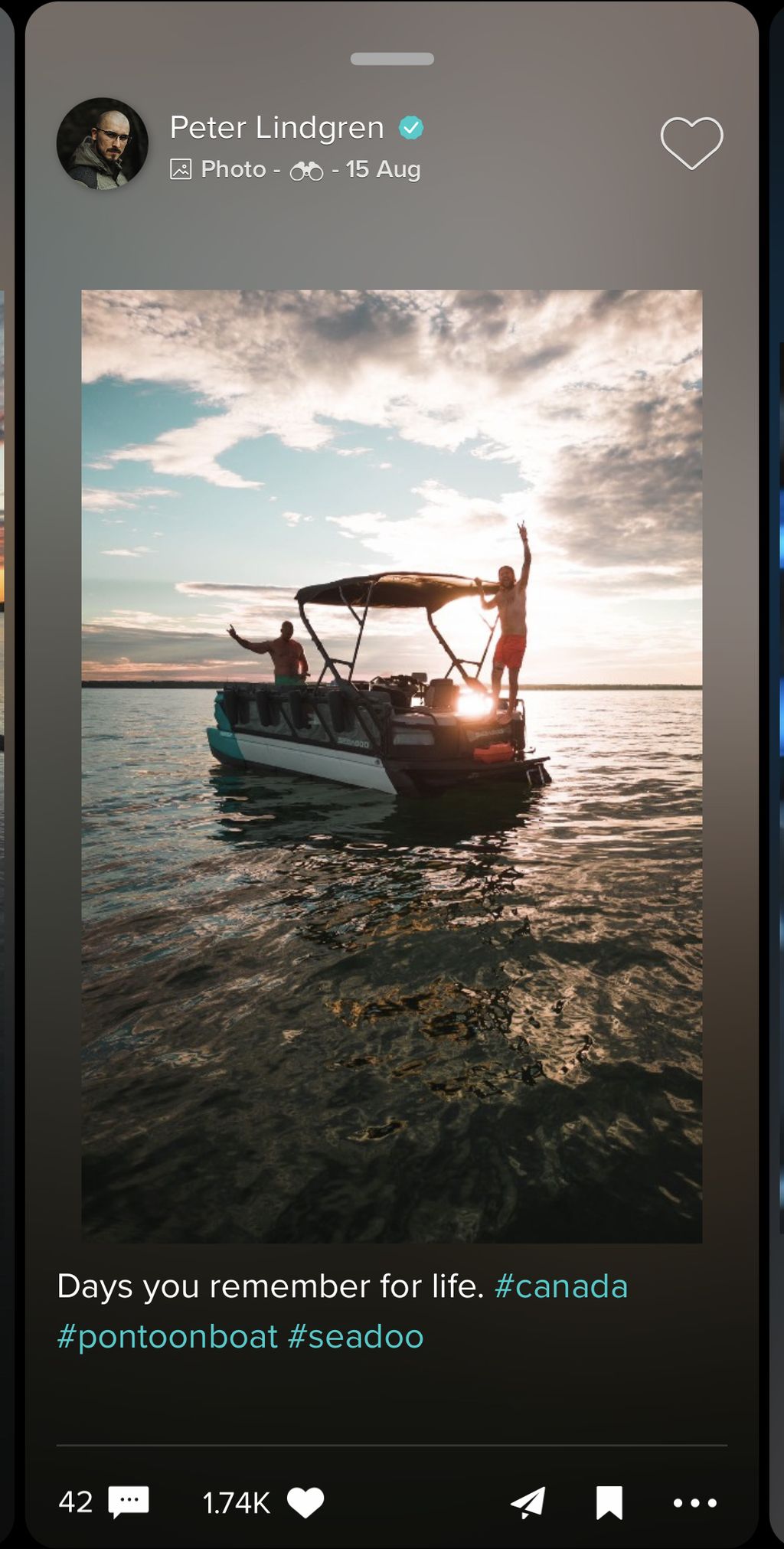In this image, we see a screenshot from a social media app showcasing a user's post. At the top, the name "Peter Lindgren" is prominently displayed, accompanied by a blue verified check symbol indicating a verified account. Below the name, the word "Photo" is shown with a binocular icon next to it, followed by the date "15 August." To the left of Peter's name, there is a profile icon depicting a man wearing glasses and a green jacket. 

On the right side of the name is an outline of a heart, presumably an option to favorite or like the profile. The main content of the post is a photo of a boat on the water with two individuals posing for the camera. The backdrop of the image features a radiant sunset, with the sun setting and the evening sky casting a warm glow over the scene.

The caption accompanying the photo reads, "Days you remember for life. #Canada #PontoonBoat #SeaDoo." The post has garnered significant engagement, with 1.74K likes and 42 comments. Additional icons are situated in the bottom right corner of the screenshot, including a direct message (DM) symbol, a bookmark, and a three-dotted line, likely for more options.